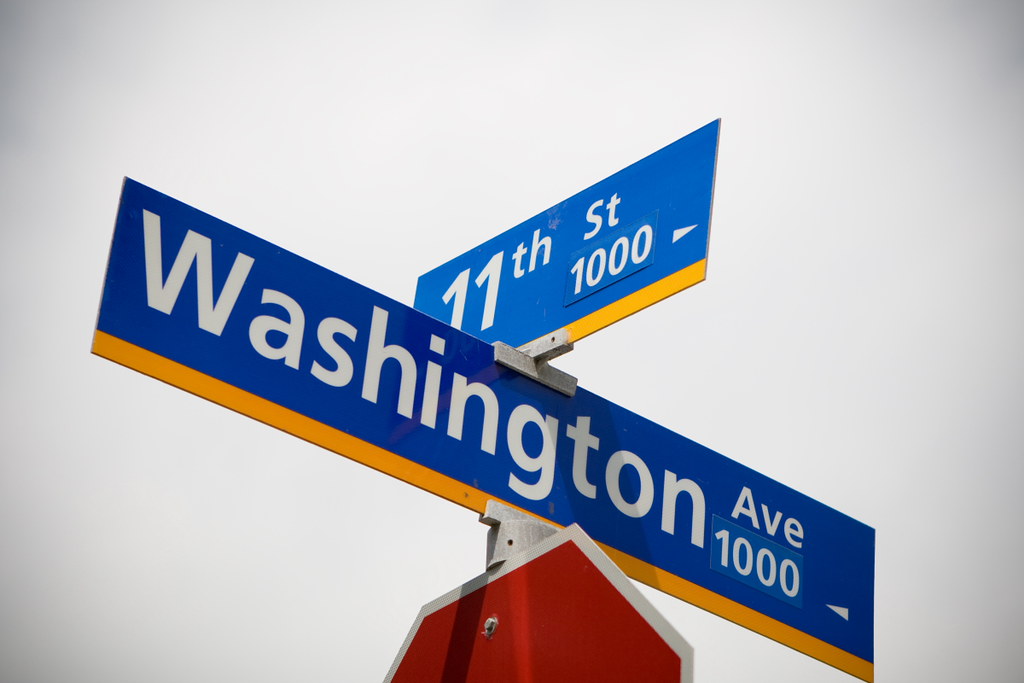The image features a trio of street signs mounted atop a stop sign. At the top, a blue street sign reads "11th St," with the number styled as "11TH," and an arrow pointing to the right. Below it, another blue sign, edged with a yellow stripe at the bottom, displays "Washington Ave," along with the number "1000" and an arrow pointing to the left. The stop sign beneath them is a classic red octagon with a bold white outline, firmly establishing the intersection's traffic control. The entire ensemble is set against a white background, with a subtle gray gradient along the edges of the photo, adding a touch of depth to the scene. Three signs are clearly visible in the image, each contributing to the navigational clarity of the urban environment.